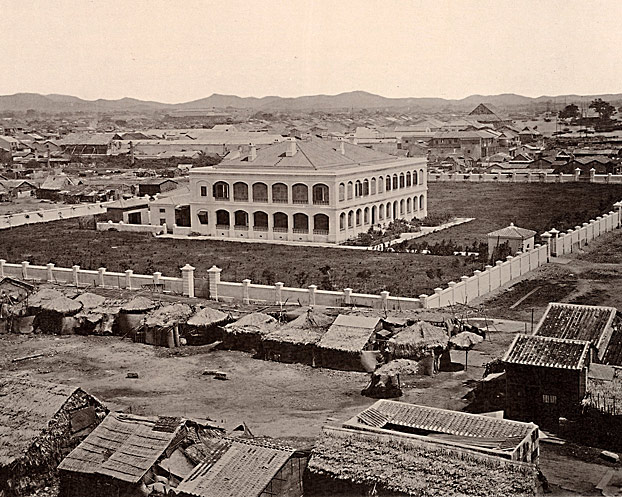This is an old black-and-white photo capturing a large, two-story building with a triangular, pointed roof and chimneys, surrounded by a sturdy white wall. The structure, possibly a wealthy person's residence, is characterized by large windows and ornate archways. The surrounding wall encloses a grassy area, starkly contrasted by the foreground and surrounding regions filled with makeshift huts constructed from wood, thatch, tarps, and plant materials. These shanty town dwellings, distributed along dirt roads, underscore the extreme poverty encompassing the opulent central building. The distant background of the image reveals a range of large, wispy, purplish mountains, further intensifying the stark disparity between the building's grandeur and the surrounding underdeveloped area.